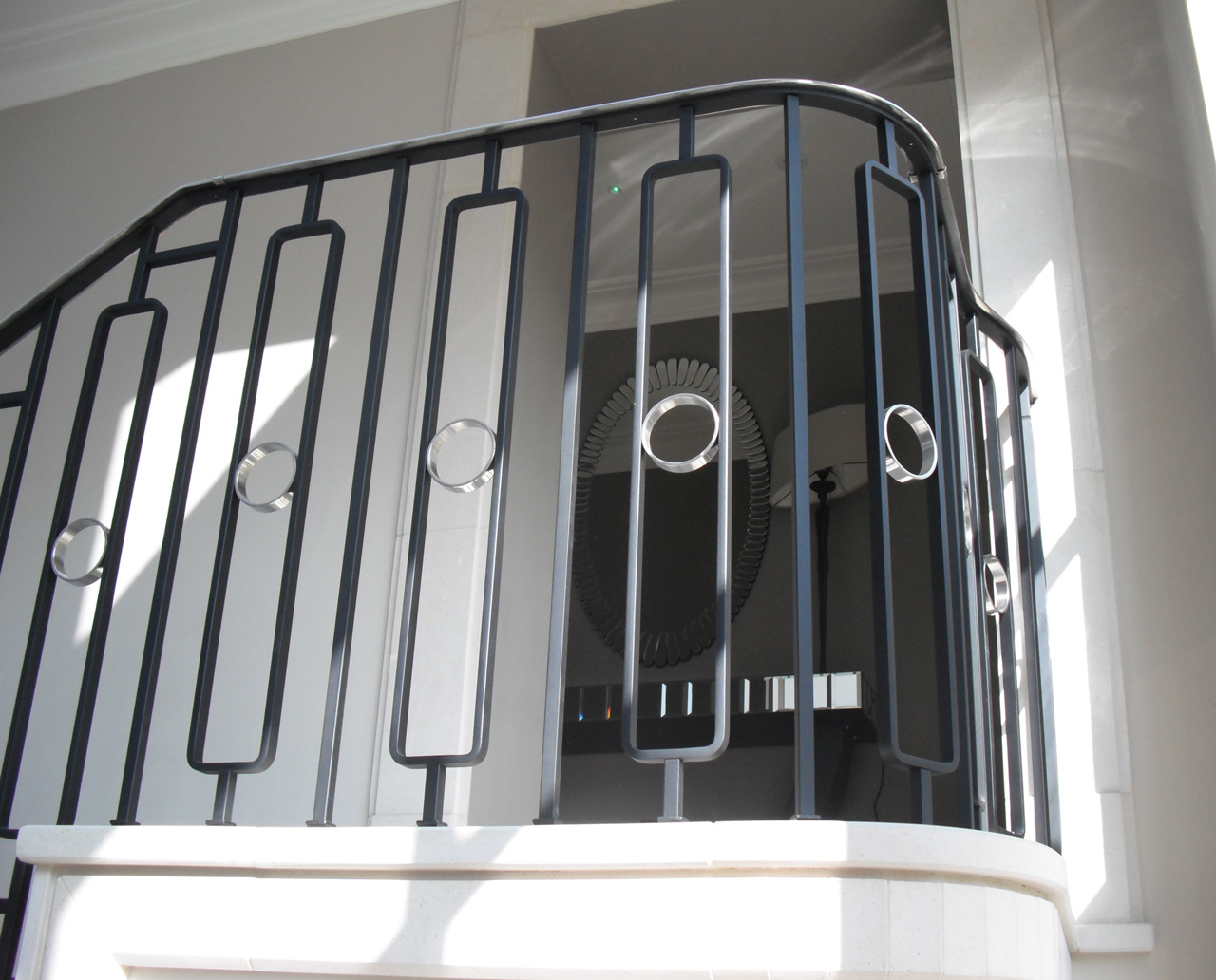The image depicts an elegant interior stairway leading to the second floor of a building. The focal point is a black metal railing with an art deco design, featuring large oblong rectangles each enclosing a small circle, spaced evenly apart by vertical poles. This railing runs along a staircase painted white, which ascends from a white, curved porch-like area. The harmonious color scheme includes light grey walls and ceiling, with white trim and doorframe accents. Adjacent to the stairway, a hallway with dark grey walls houses a sophisticated oval mirror, bordered by small rectangular details, adding to the style of the décor. Beneath the mirror sits a reflective silver side table, adorned with a sleek, shiny table lamp. The cohesive design elements and fine details suggest a beautifully designed, elegant home interior.